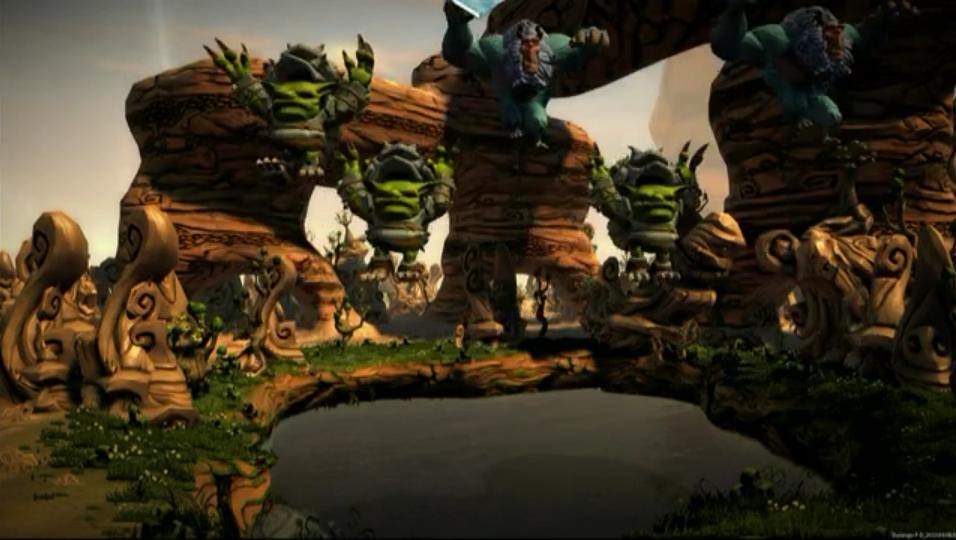The image, likely a video game still, depicts a dark, fantastical landscape characterized by intricate rock formations and a hint of otherworldliness. Dominating the foreground is a black, oval-shaped pond encircled by tan rocks interspersed with patches of grass. On the left side, three elaborately carved statues with French curves stand amidst the terrain, somewhat resembling alien musical notes.

In the center of the image, three lime-green, goblin-like creatures are captured either falling or leaping into the air, their oversized hands—each with three fingers—outstretched above their heads as though partaking in some eerie ritual. Alongside them, a monkey-like figure dressed in a blue spandex suit and sporting white facial hair mimics their pose. Behind them, a curved arch formation with a flat top stands, hinting at the ancient, mysterious nature of this landscape.

Adding to the surreal tableau, two large, dark blue humanoid figures flank the scene, both vaguely ape-like and appearing to hold something in their right hands. The right side of the image is cloaked in shadow, heightening the sense of danger and secrecy on this enigmatic island. The entire composition evokes an atmosphere of ancient peril, hidden treasures, and mythic creatures, making it a quintessential setting for an epic video game adventure.